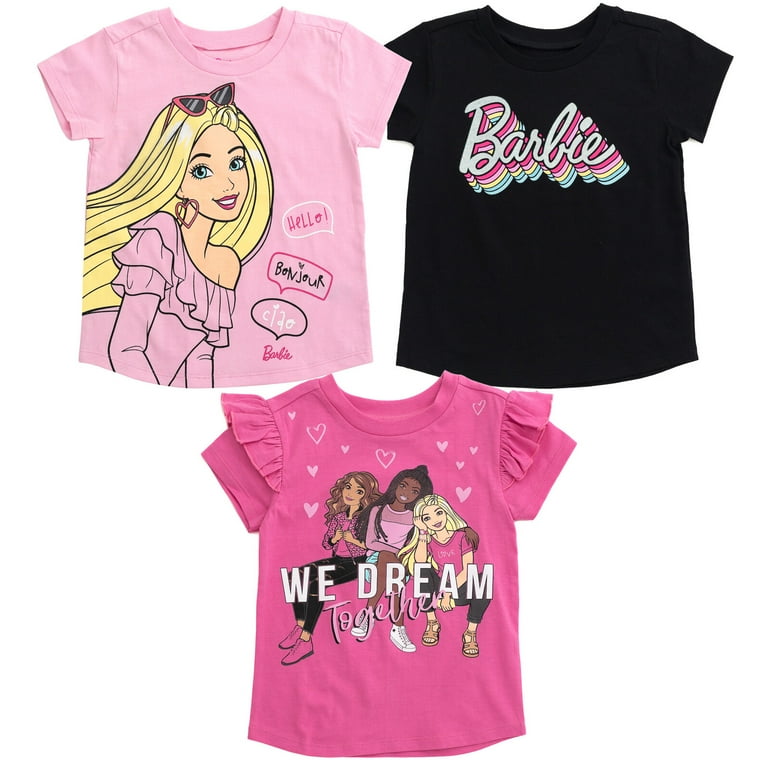This image features a set of three Barbie-themed t-shirts for young girls, presented in an appealing layout. At the top left, there is a pink crewneck t-shirt adorned with a detailed illustration of Barbie. Barbie is depicted with long blonde hair, red-framed sunglasses perched on her head, heart-shaped earrings, and she wears an off-the-shoulder ruffled pink dress. Surrounding her are three speech bubbles saying "Hello," "Bonjour," and "Ciao," with the name "Barbie" inscribed below in pink cursive.

Adjacent to this, on the top right, is a black short-sleeved t-shirt. This shirt features the word "Barbie" prominently displayed in cursive with a multicolored pastel shadow effect, incorporating hues like purple, violet, yellow, green, and blue.

Positioned below these, in the center, is a darker pink t-shirt with frilly shoulder details. The t-shirt is decorated with numerous white hearts near the collar and showcases a vibrant cartoon illustration of three girls—two of them light-skinned and one dark-skinned. These girls are depicted sitting close together, surrounded by hearts, and the words "We Dream Together" are printed across their legs.

Each t-shirt combines classic Barbie imagery with modern design elements, making them ideal for young preteen girls.